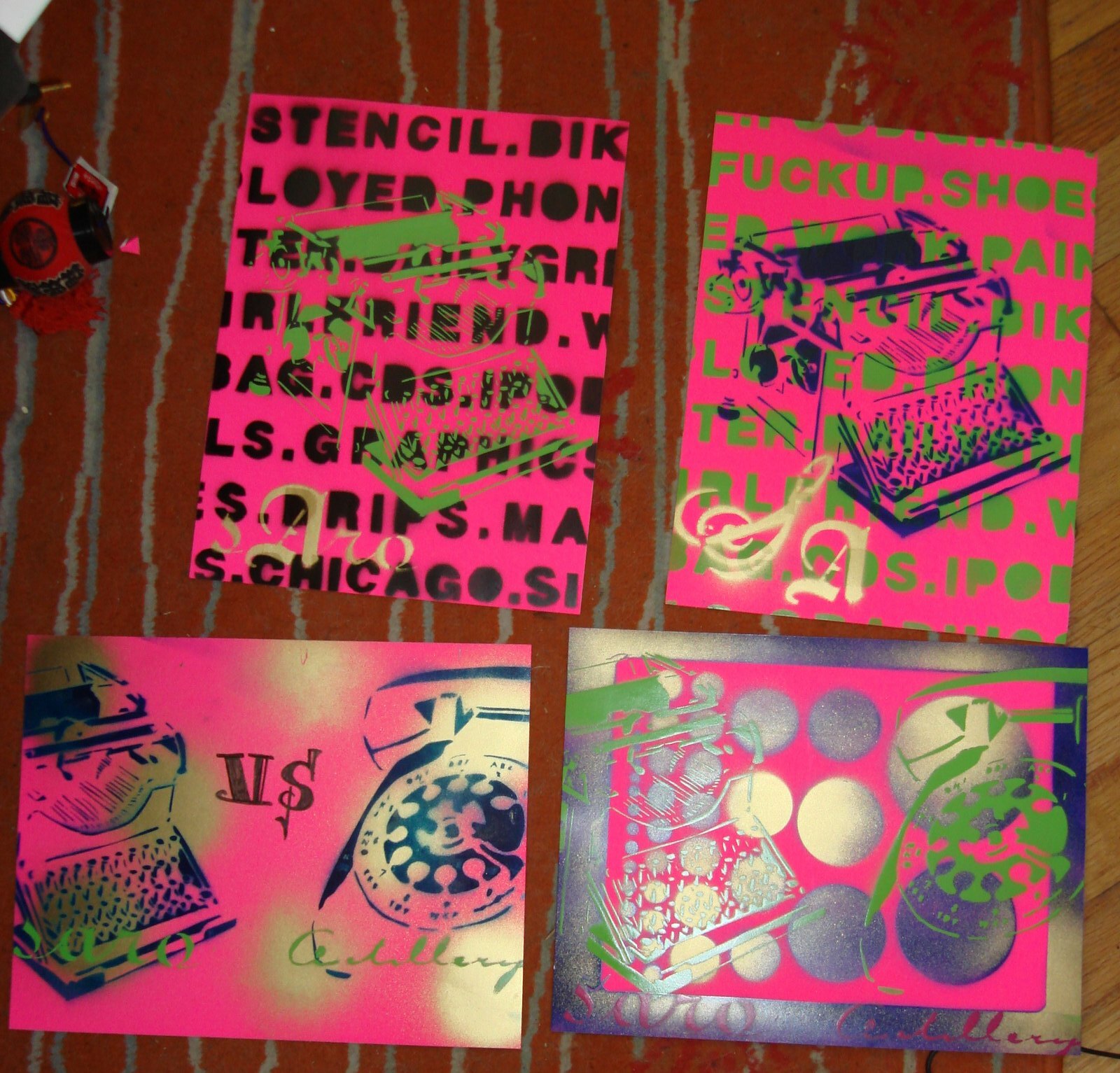This is a photograph featuring four small, poster-like sheets of paper, arranged on a vibrant, red background with a green drizzle pattern. The overall theme is dominated by pink and includes recurring images of old mechanical typewriters. The top two sheets are positioned in a portrait orientation and are slightly tilted to the right, while the bottom two are landscape-oriented. The top left sheet prominently displays the words "Stachel Bic Lloyd," although some text is cut off at the edges, creating a fragmented look. The top right sheet features the phrases "Fuck Up Shoe Pain" along with other partially obscured text. The bottom left sheet showcases a typewriter and a rotary phone, juxtaposed in a visually striking manner, while the bottom right sheet contains illustrations of balls. The background field of each sheet varies, with some displaying green dots and others blue and white dots, adding to the visual complexity. In addition, some sheets have stenciled words such as "stencil," "drips," and "graphics," giving the whole collection a dynamic and layered appearance. The image is complex and vivid, with the apparent use of airbrushing and bright neon colors adding to its eclectic aesthetic.